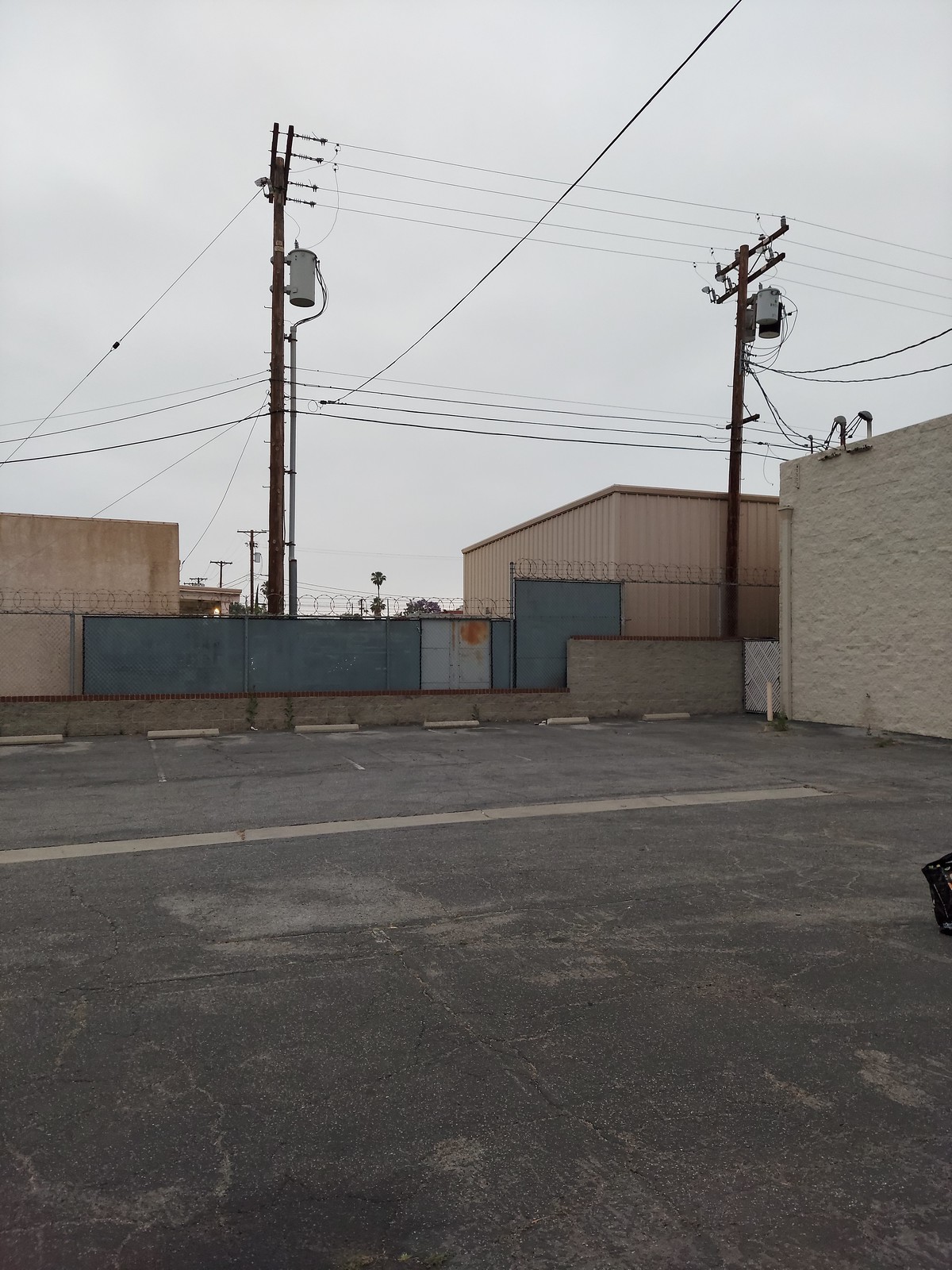The photograph, oriented vertically, captures a bleak and utilitarian industrial area. Dominating the foreground is a large, vacant parking lot with diagonal parking spaces delineated by concrete barriers to prevent vehicles from colliding with the fence. The lot is devoid of cars, further enhancing the desolate atmosphere. 

Stretching from the left to the right and partially obscuring the sky, a network of telephone wires hangs between sturdy poles—two of which can be seen in the middle distance. One particularly long wire cuts a path from the lower left to the upper center of the image, drawing the eye upward.

A chain-link fence borders the parking lot, its upper edge looped and topped with coverings in varying shades of gray, effectively blocking the view beyond. Behind the fence, three cube-like, rectangular-shaped industrial buildings loom. Their tannish-brown exterior walls give them a utilitarian and somewhat weathered appearance. The building on the left appears modest in size, while the one on the right is either foreshortened or larger. Another similar structure is situated within the bounds of the parking lot itself.

The landscape is punctuated by palm trees in the background, suggesting that this industrial area resides in a region with a warmer climate. The overall scene is stark and uninviting, capturing the raw, functional essence of an industrial zone.